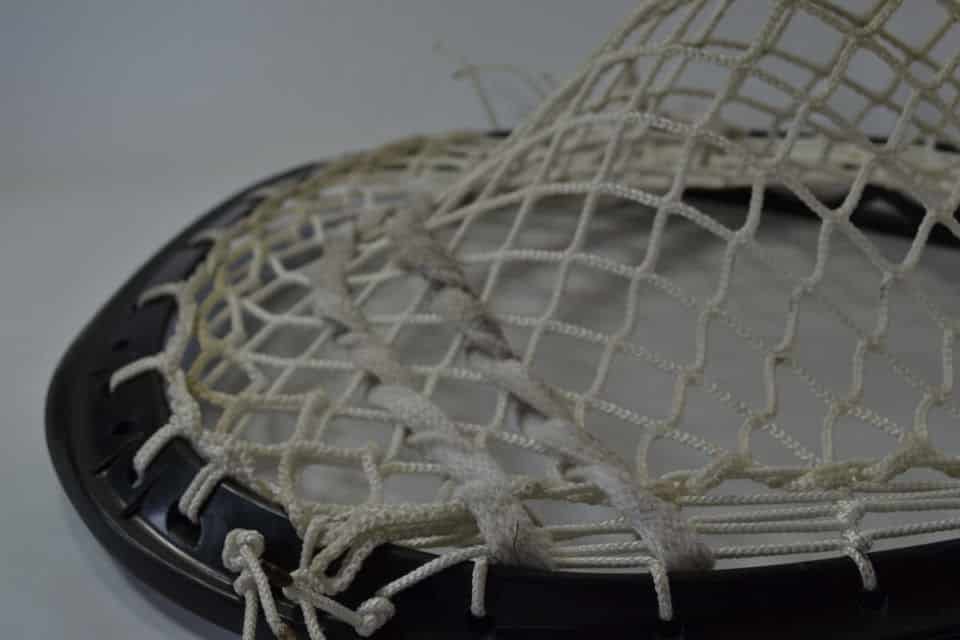The image depicts a large, close-up view of a net, most likely part of lacrosse equipment. The black hard plastic hoop, which the net is bound to, is positioned towards the right side of the image and extends into the middle. The net itself features diamond-shaped mesh tied tightly around the frame, with additional strings lacing across to reinforce it. Slight green stains on the netting suggest usage, possibly on grass. The net rests on a solid white surface, possibly a table, with minimal illumination highlighting shades of black, white, and gray in the composition. Two ropes are visible, securing the net in place and preventing it from flexing fully, with a potential handle clipping at the far right edge.